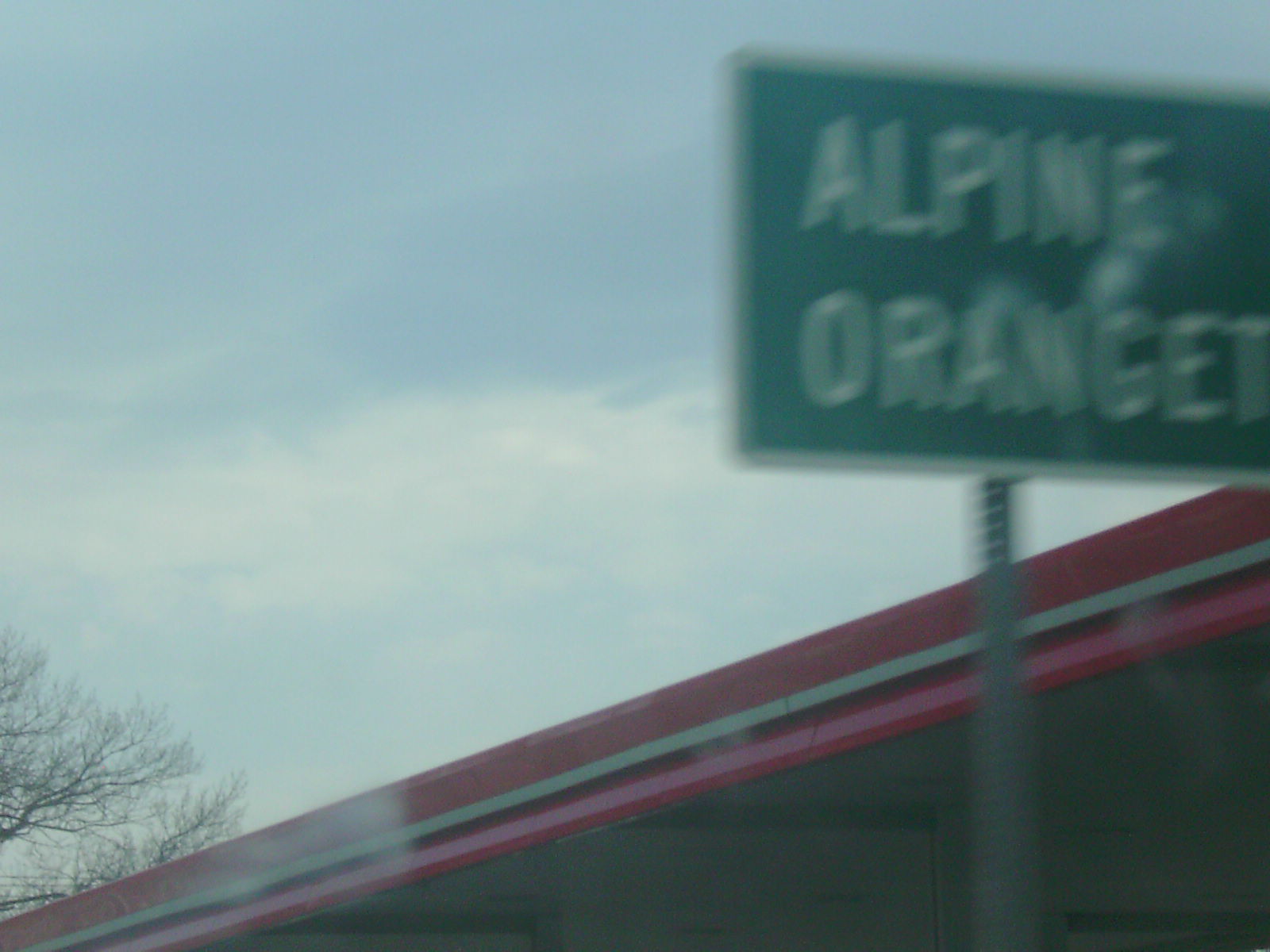A clear blue sky dotted with fluffy white clouds serves as the backdrop for this vibrant scene. On the left side of the image, a dormant tree with bare branches stretches upwards, devoid of any leaves. To the far right, green text reading "Alpine Orchid" is prominently displayed against a similarly green background. Below this text, a marabou can be seen, providing a touch of wildlife to the setting. Dominating the lower portion of the image is the canopy of a building, adorned with purple and white lines interspersed with black stripes, and tinged with slightly pink hues towards the bottom. The entire scene has a dreamy quality, as if viewed through a glass barrier, adding an ethereal touch to the photograph.